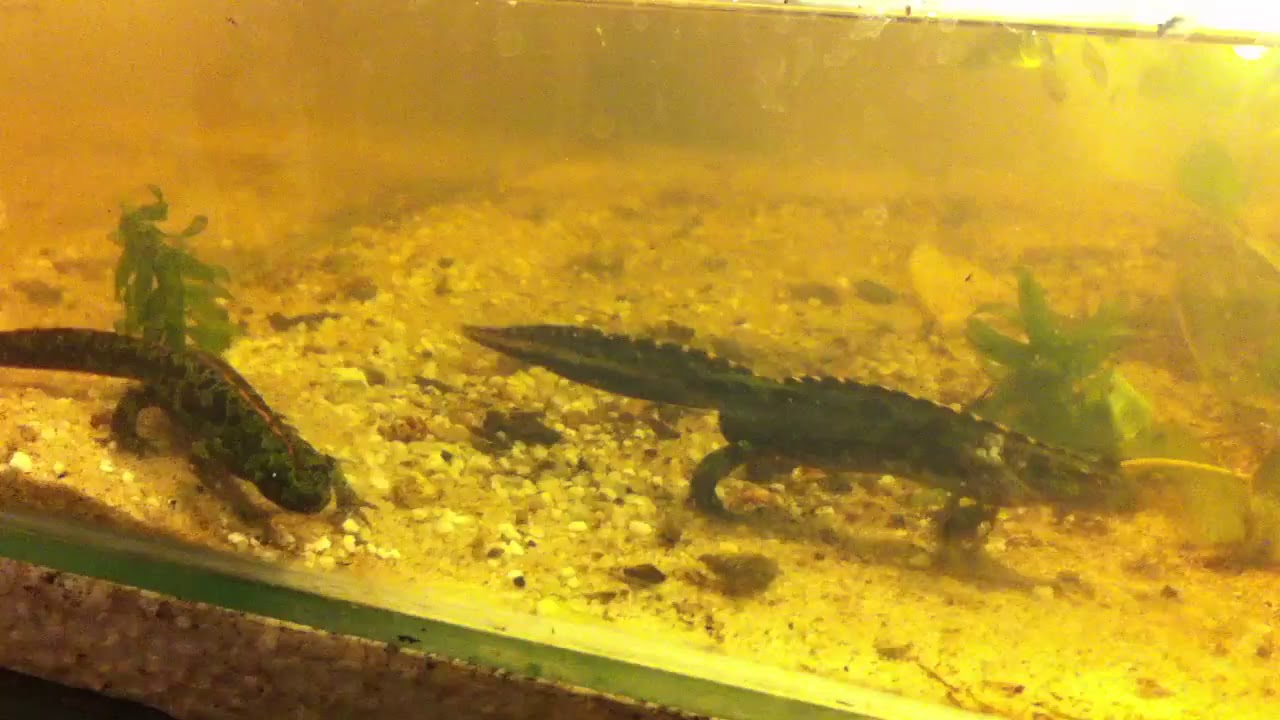This photograph captures the interior of a glass aquarium with a yellowish tint. Inside the aquarium, the slightly muddy water reveals a floor covered with a mixture of white, black, and brown pebbles. Two amphibians, possibly newts or salamanders, are featured prominently. They have dark green bodies adorned with black spots, long tails, and distinctive spiny ridges running along their backs and tails. These creatures, crawling on all fours, are surrounded by patches of green vegetation. One amphibian is oriented towards the right while the other faces the camera. The scene is bathed in a yellowish light, suggesting the presence of a heat lamp overhead.